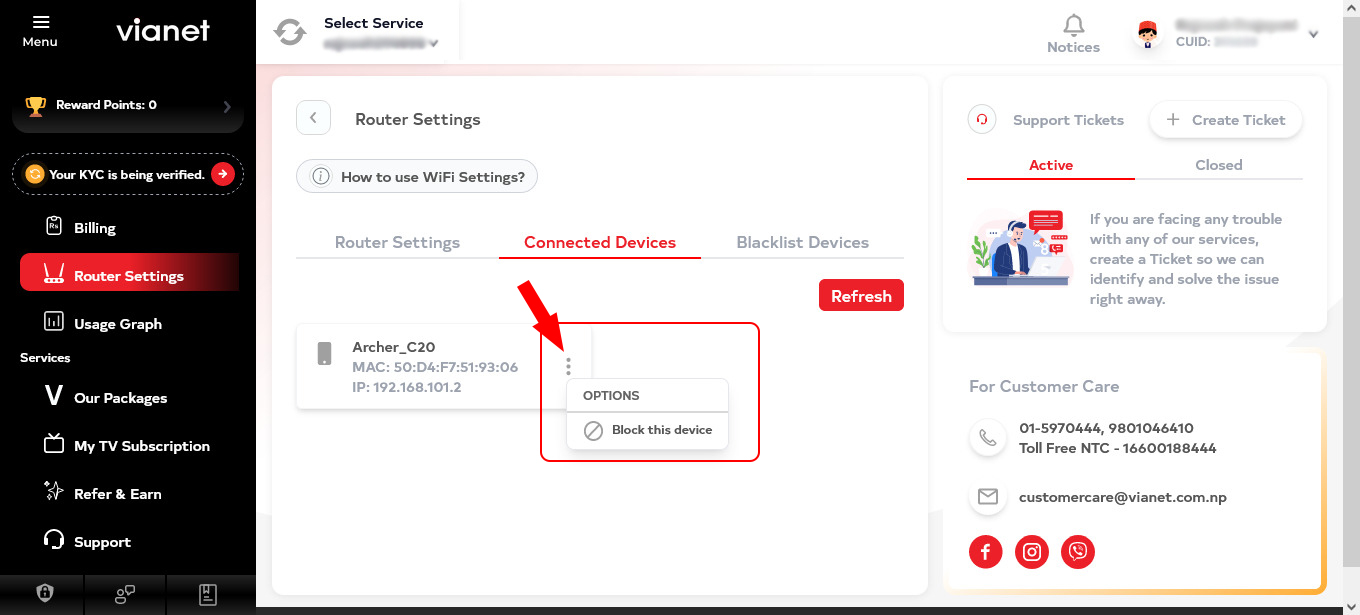The image showcases the user interface of a technology-focused website, likely associated with an internet and TV service provider named "Vianet". The layout is distinctly horizontal and rectangular. On the left, occupying approximately 15-20% of the space, is a solid black sidebar featuring a menu. At the top of this sidebar is the "Vianet" logo, followed by a series of options: "Reward Points," "Your KYC is being verified," "Billing," "Router Settings," "Usage Graph," "Services," "Our Packages," "My TV Subscription," "Refer and Earn," and "Support." The "Router Settings" option is highlighted in red, indicating it is currently selected.

To the right of the sidebar is the main content area, filling about half of the screen. This section is labelled "Router Settings" and includes a list of submenu options: "Select Services," "Router Settings," "How to Use Wi-Fi Settings," and "Connected Devices," with the latter being highlighted.

To the left of this section, under the "Router Settings" heading, are options related to managing devices, including "Blacklist Devices". Beneath these options is a "Refresh" button. Additionally, detailed below this is information about a specific device—the "Archer C20," displaying its MAC address and IP address, along with an option to block the device.

On the far right, another section labelled "Notices" and "Support Tickets" allows users to create a ticket or check the status of existing tickets, categorized as "Active" or "Closed." Contact information is provided for further assistance, listing both a regular and a toll-free customer care number, along with a customer service email address: customercare@vnet.com.np. Social media icons, including one for Instagram, suggest additional ways to reach customer support.